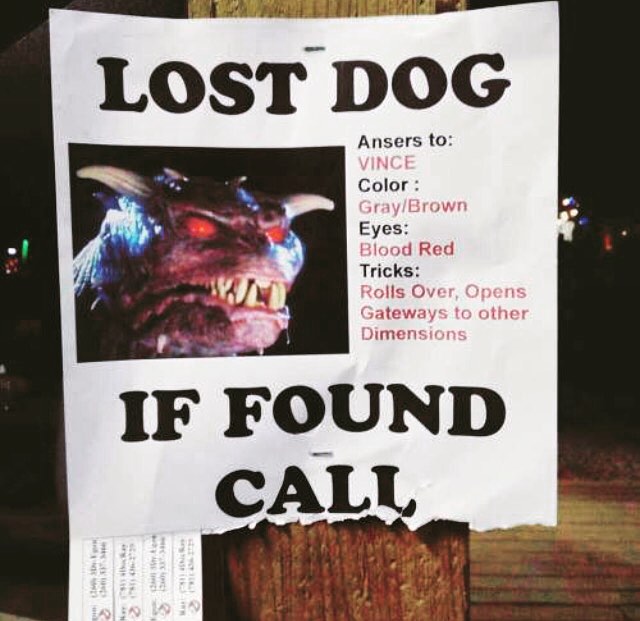A humorous and eerie "lost dog" poster stapled to a telephone pole in a dimly lit area with a black background and a few visible lights. The top of the white printed sign reads "LOST DOG" in bold letters. Below the text, instead of a typical dog photo, there's an image of a monstrous creature with horns, blood-red eyes, sharp teeth, and drool. To the right of this unsettling picture, the text reads: "Answers to: Vince. Color: Gray-Brown. Eyes: Blood Red. Tricks: Rolls over, opens gateways to other dimensions." Below these details, it says "If found, call," followed by four tear-away pieces with contact numbers, though most of them have already been removed.